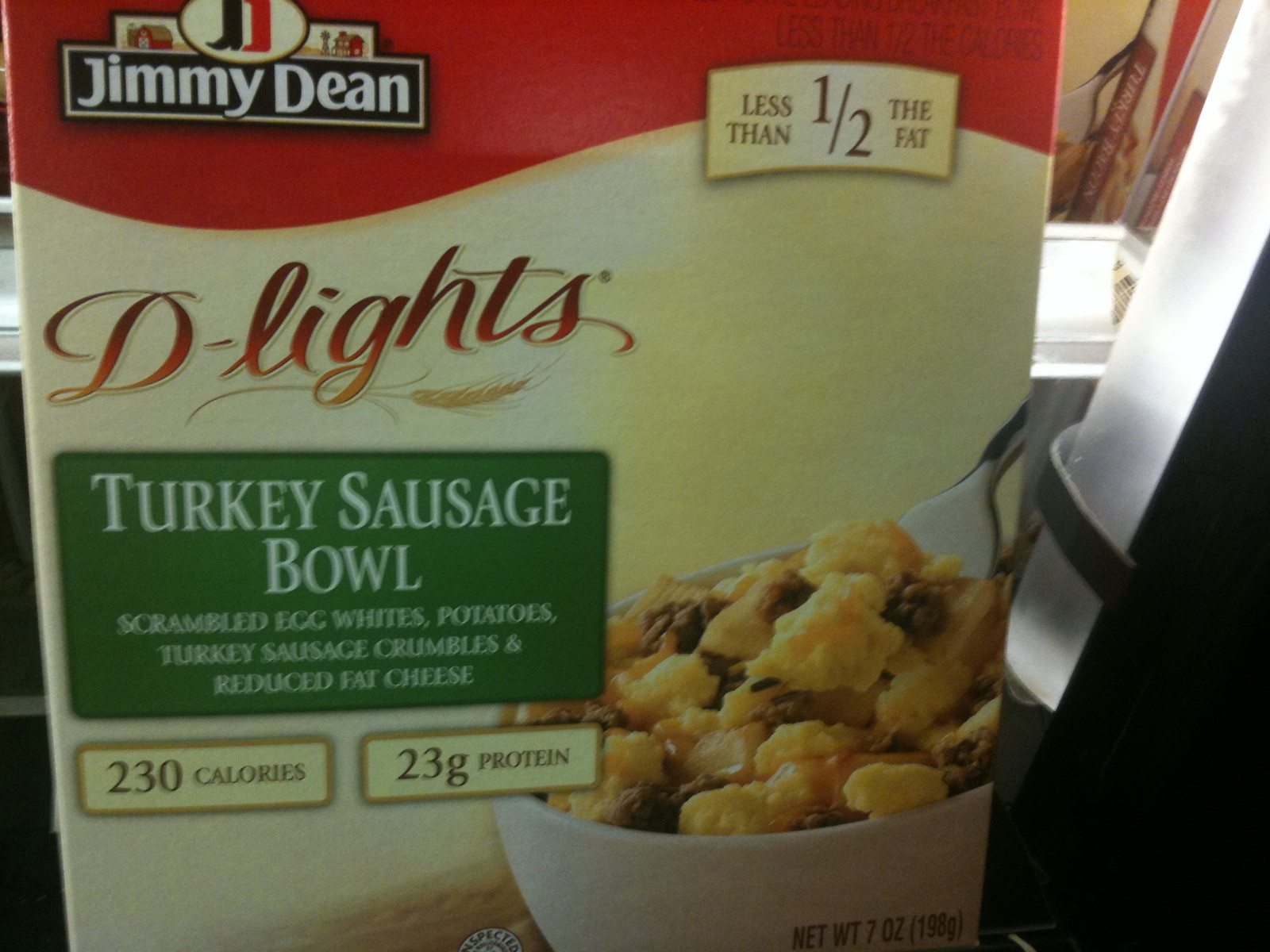This close-up color photograph depicts a Jimmy Dean D-lights Turkey Sausage Bowl packaged food product. The top left corner features the Jimmy Dean logo, with "Jimmy Dean" written in bold white lettering against a black background, encased in an off-white trim. Above the logo, there appears to be an oval with a small image, possibly a red barn and another building. To the right of the logo, the package claims "less than half the fat." Directly below, the product name "D-lights" is prominently displayed in a script font, with the "D" as a large capital letter followed by a hyphen and "lights" in brownish to tan gradient lettering. 

Below the D-lights branding, a green rectangular area contains the text "turkey sausage bowl" in all capitalized white letters. The ingredients list below this includes "scrambled egg whites, potatoes, turkey sausage crumbles, & reduced fat cheese," also in capitalized white letters. To the right of the ingredient list, there are two small cream-colored rectangles with a golden border; one states "230 calories" and the other "23g protein." 

The right half of the box displays a white bowl containing the food product. The bowl shows scrambled egg whites, browned turkey sausage crumbles, potatoes, and cheese, with a silver fork visible inside, scooping a portion of the food. The handle of the fork extends off the right side of the image. The overall color scheme of the box includes red at the top, blending into a cream-colored background where the product details are listed. The background also contains some indistinct elements like a bright fluorescent light and possibly other objects in the distance, partially visible behind the box.